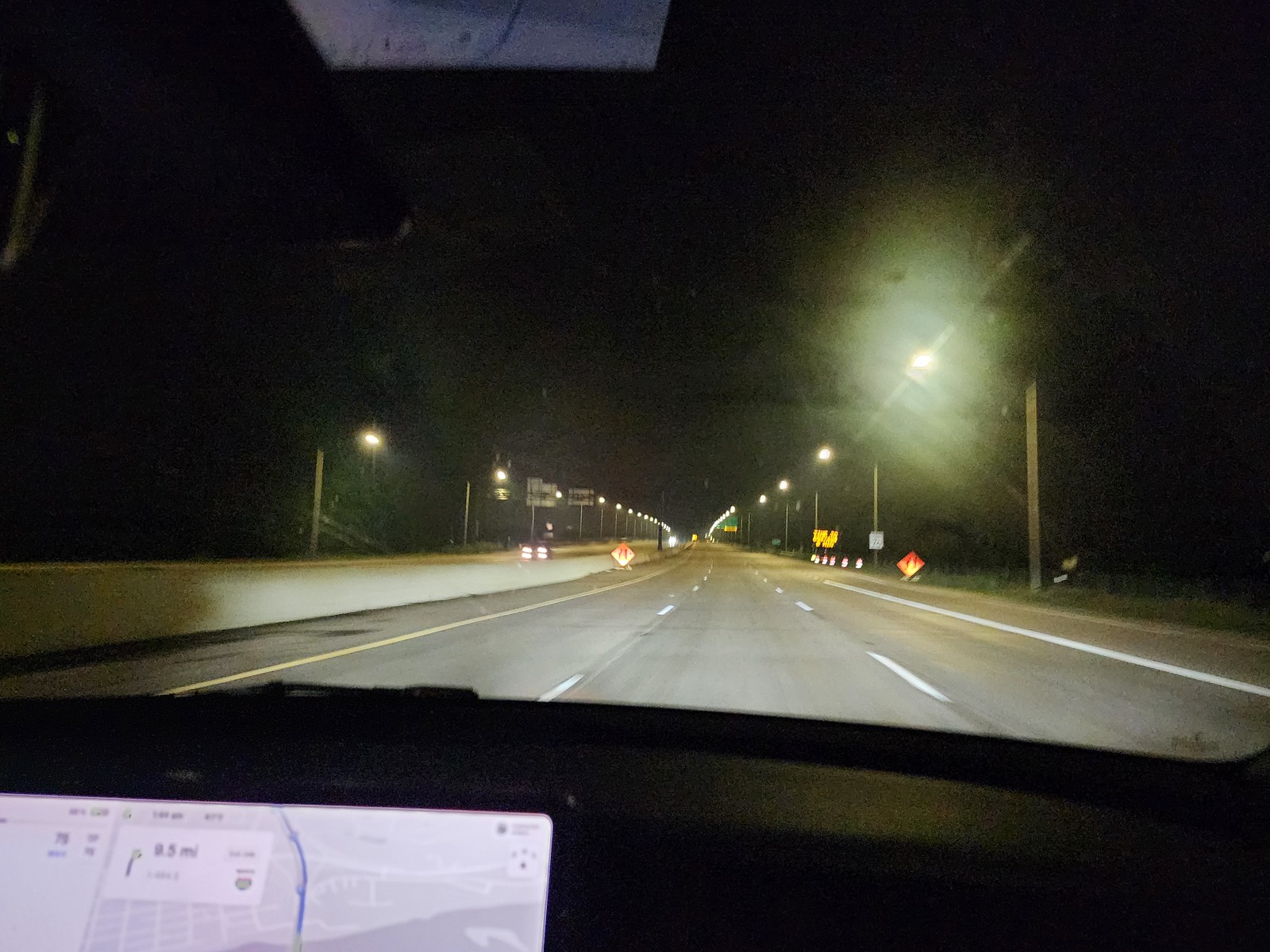A captivating night-time photograph depicts the interior of a car from the perspective of the dashboard, offering a unique and intimate view of the street ahead. The inky black sky is punctuated by street lamps lining both sides of the road, casting pools of warm light that illuminate the street in a rhythmic pattern. Within the car, the navigation system glows softly in the lower left-hand corner of the image, providing a subtle but essential guide for the driver. On the street, an orange warning sign is visible on the right side, accompanied by a strip of grass that adds a touch of greenery to the scene. An additional orange sign stands on the left side of the road, near an electronic signboard displaying vital information for motorists. The combination of elements creates an evocative snapshot of a night drive, blending the technological with the natural and the necessary with the ambient.